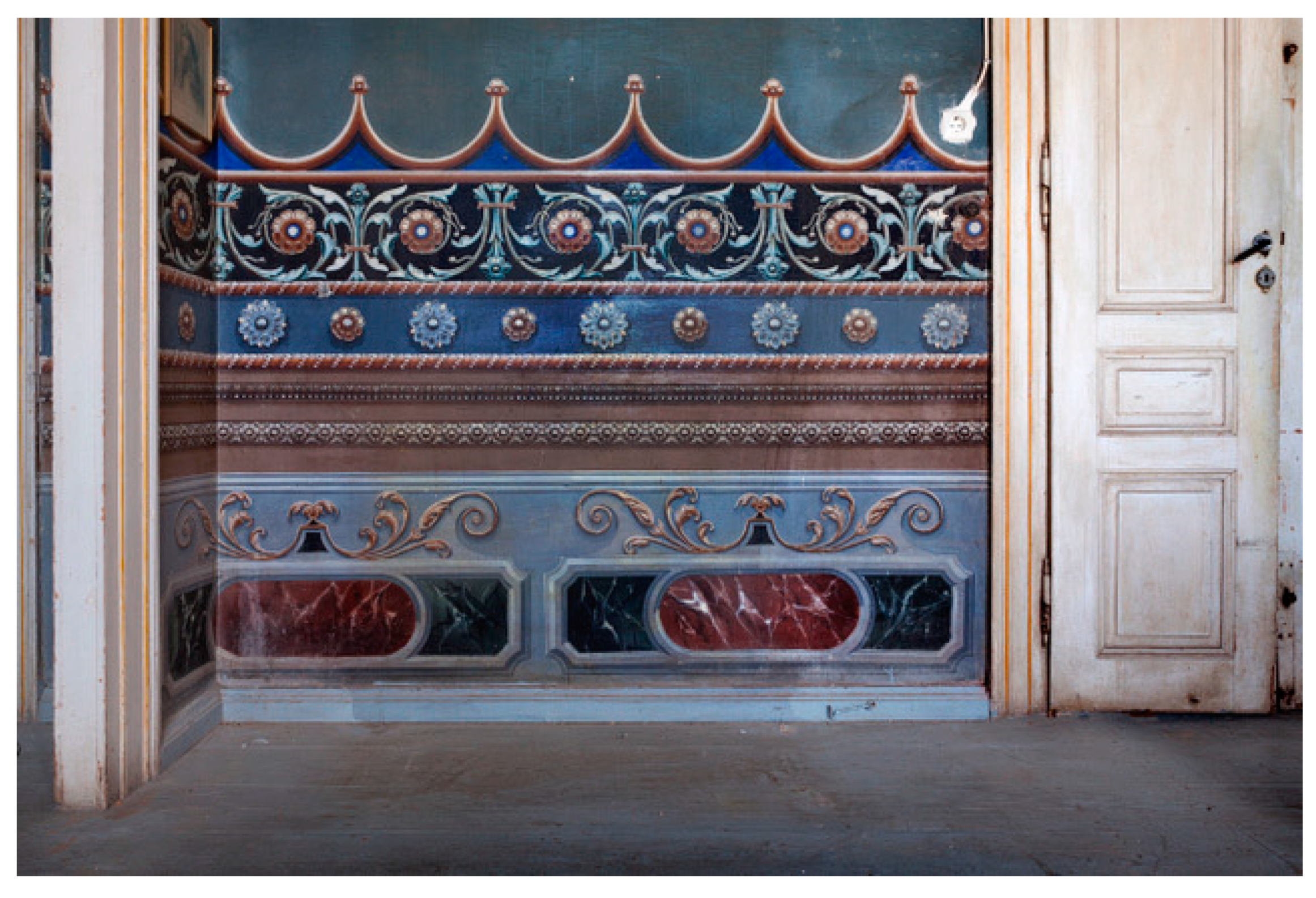The photograph captures an older, possibly abandoned house featuring a prominently detailed wall and a narrow, aging door on the right side. The white or cream-colored door, now dirty and discolored, includes an old-fashioned lock and hardware indicative of a bygone era, further suggesting the house's age. The wall is adorned with an ornate, intricate mural or wallpaper in vibrant shades of emerald, jade, blue, and gold, interspersed with red and green accents. 

At the top of the wallpaper, there is a scalloped pattern resembling ocean waves, outlined in gold with a blue interior. This is followed by several distinctive decorative bands: one with floral rose detailing amidst green foliage, another blue stripe with red and blue flowers, and additional sections highlighted by brown, gold, and white designs. A notable feature is a band resembling rope lines interspersing round medallion patterns on a blue background, concluding with intricate gold scrollwork against a pale blue backdrop with panels of dark green and dark red, giving a marble-like effect.

The door frames are notably dirty and faded, with peach stripes painted vertically along their sides. This elaborate detailing on the wall, along with the weathered appearance of the door and frames, emphasizes the building's antique character and uninhabited state. The flooring beneath this vivid wall could be plain wood or cement, contributing to the overall tired and neglected ambiance of the room.